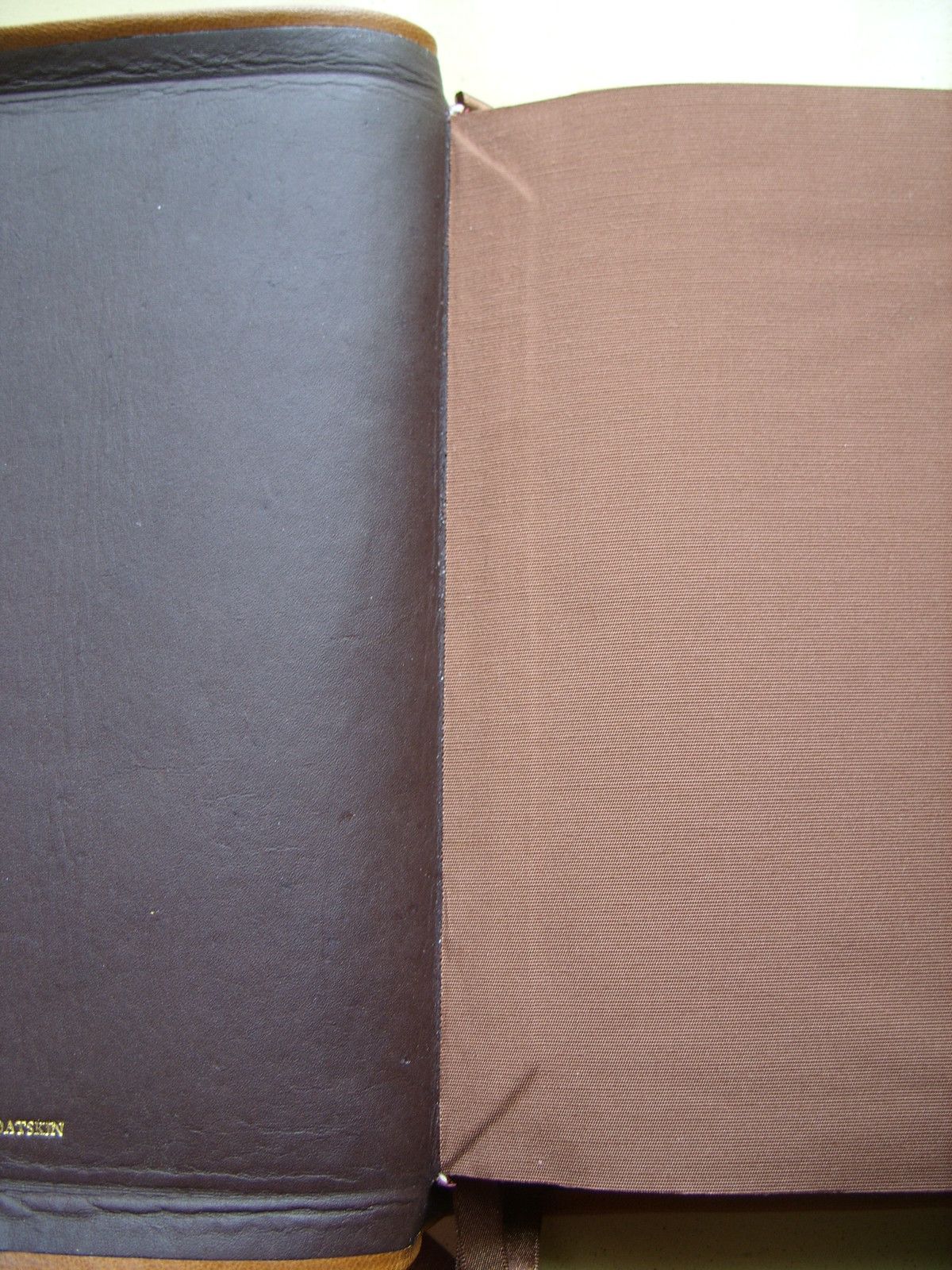This photograph features a detailed close-up of a folded leather-bound item, appearing to be a book, likely a Bible. The left side of the image displays a silver-blue, gray-trimmed zippered case with brown accents on the top and bottom. Gold lettering is inscribed on the lower part of this section. The right side of the photo reveals a reddish-beige or rose pink insert or exterior, possibly made of linen, with a canvas-like texture, folded around a thin rod, and stitched or glued to itself. Both sections appear to be standing on their edges against a white background, with the gray item including small engraved letters in gold on the lower left corner. The complex binding and additional fabric that folds over the leather case further suggest it is a high-quality book cover, reinforcing the impression that this is a photograph of a folded Bible.